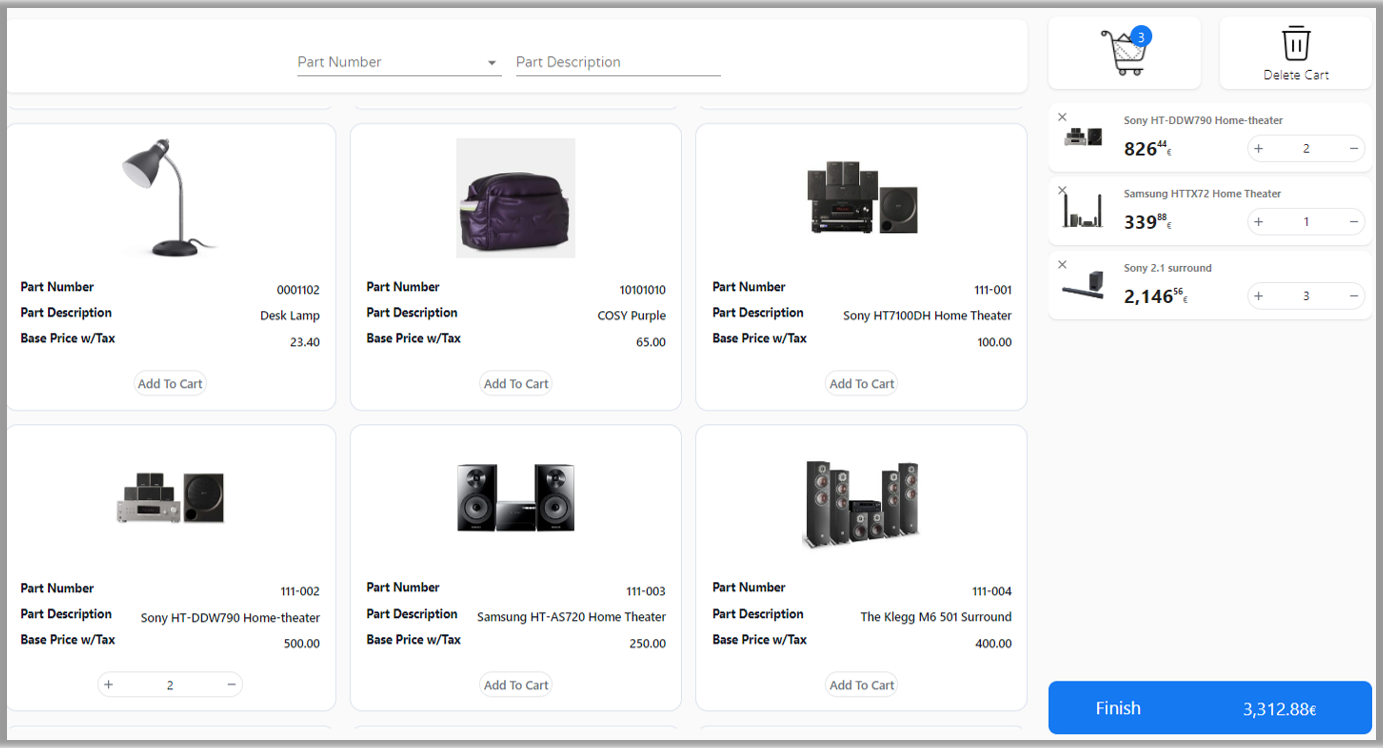Screenshot of a website showcasing various items for sale. At the top of the page, there's a header displaying "Part Number" along with a dropdown menu and "Part Description." To the right, a shopping cart icon reveals that there are three items currently in the cart; a "Delete Cart" button is also present.

The main section features a grid of items in two rows. The items in the top row from left to right are a lamp, a bag, and a home theater system. The bottom row, in the same order, shows another home theater system, a Samsung home theater system, and a surround sound system.

The shopping cart summary displays the following items:
1. Home theater system priced at $826.44 with a quantity of 2.
2. Another home theater system priced at $339 with a quantity of 1.
3. Surround sound system priced at $2,146.16 with a quantity of 3.

There is no visible company branding on the website, making it unclear which retailer operates this site.